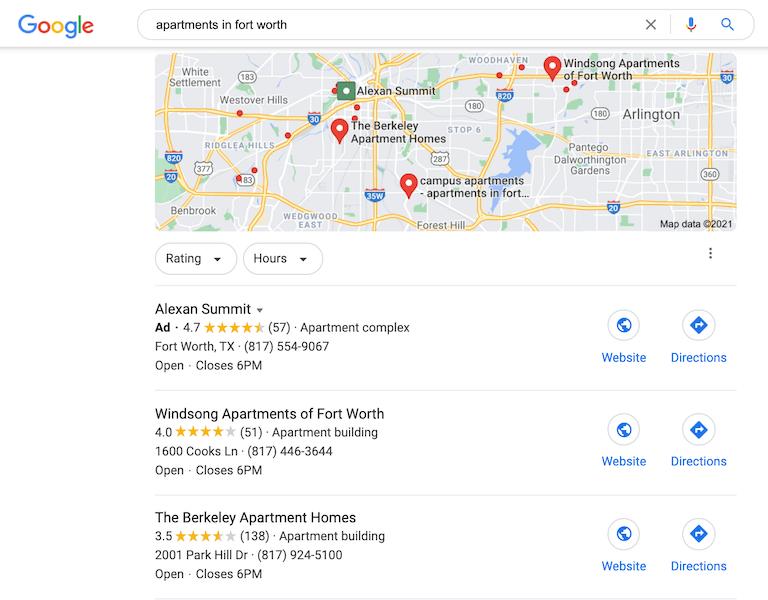The image depicts a Google search results page for "apartments in Fort Worth." At the top is the Google search bar with the query entered. The interface includes a microphone icon, a magnifying glass (search button), and an 'X' for clearing the search.

Below the search bar is a map of Fort Worth, showcasing the locations of different apartment complexes identified in the search. Beneath the map, the first search result appears as a sponsored ad for "Alexan Summit," boasting a rating of 4.7 stars based on 57 reviews. It’s noted as an apartment complex situated in Fort Worth, Texas.

The second listing features "Wind Song Apartments of Fort Worth," with a 4-star rating and 51 reviews. Following this, the third listing presents "The Berkeley Apartment Homes," which has a rating of 3.5 stars from 138 reviews.

Each apartment listing includes blue action buttons labeled "Website" and "Directions," facilitating quick access to more information and navigational assistance. The listings are complemented by an icon next to these action buttons.

Above the list of search results, two drop-down menus allow users to filter the results by ratings and hours of operation. All these controls collectively enable a streamlined process for sorting and refining the apartment search. The map on the page also visually indicates the locations of "The Berkeley Apartment Homes" and "Wind Song Apartments," aiding the user in geographical orientation.